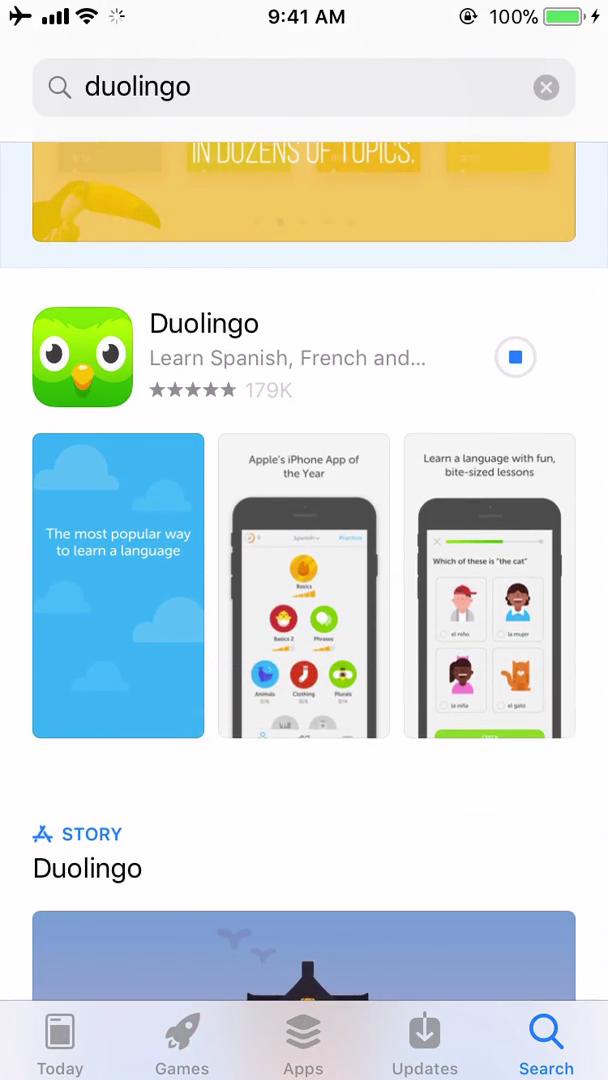A detailed screenshot showcases a typical Android device interface. At the very top of the screen, you can see a series of status icons, including an airplane icon indicating airplane mode is active, signal strength bars, a Wi-Fi signal indicator, and a small rotating icon signifying ongoing data activity. The upper right corner shows the time as 9:41 AM, while the upper left corner features a lock icon, battery strength, and a charge bolt indicating the battery is currently charging.

Below this status bar is a gray search box with the word "Duolingo" typed into it, suggesting the user is searching for this application. Beneath the search box, the layout resembles an app store or Google Play Store, displaying various app sections. A partially visible, chopped-off yellow banner likely represents an advertisement.

Prominently featured in the middle of the screen is the Duolingo app listing, displaying the recognizable green owl icon on the left. The app listing includes a brief description, "Learn Spanish for...", followed by an ellipsis. It also shows the app's high rating of five stars and the number of reviews, totaling 179K. 

Directly below this app listing, there are three illustrative screenshots offering a preview of Duolingo's features. Further down the screen, there is a story section titled "Duolingo." This section includes a banner that is unfortunately cut off, preventing the full content from being visible.

At the very bottom of the screenshot, a gray navigation bar displays categories such as "Today," "Games," "Apps," "Updates," and "Search," with "Search" highlighted in blue, indicating the active section of the app store interface.